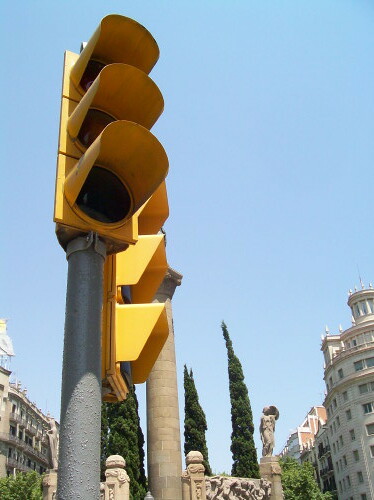The image captures a pair of distinctive yellow traffic stoplights mounted on metal poles. These lights, characterized by yellow-painted housings, feature both rounded and square protective covers over the non-illuminated red, yellow, and green lights. The traffic lights are oriented at different angles: one faces slightly towards the bottom right corner, while the other directs straight to the right. The scene is set against a backdrop of an old cityscape, reminiscent of European architecture, complemented by well-manicured trees and various signs also encased in yellow metal, potentially signaling pedestrian or cautionary instructions. In the background, there is a mixture of high brick and stone buildings, a column, and statues, suggesting a quaint town square or courtyard. All of this is enveloped in a serene light blue sky.